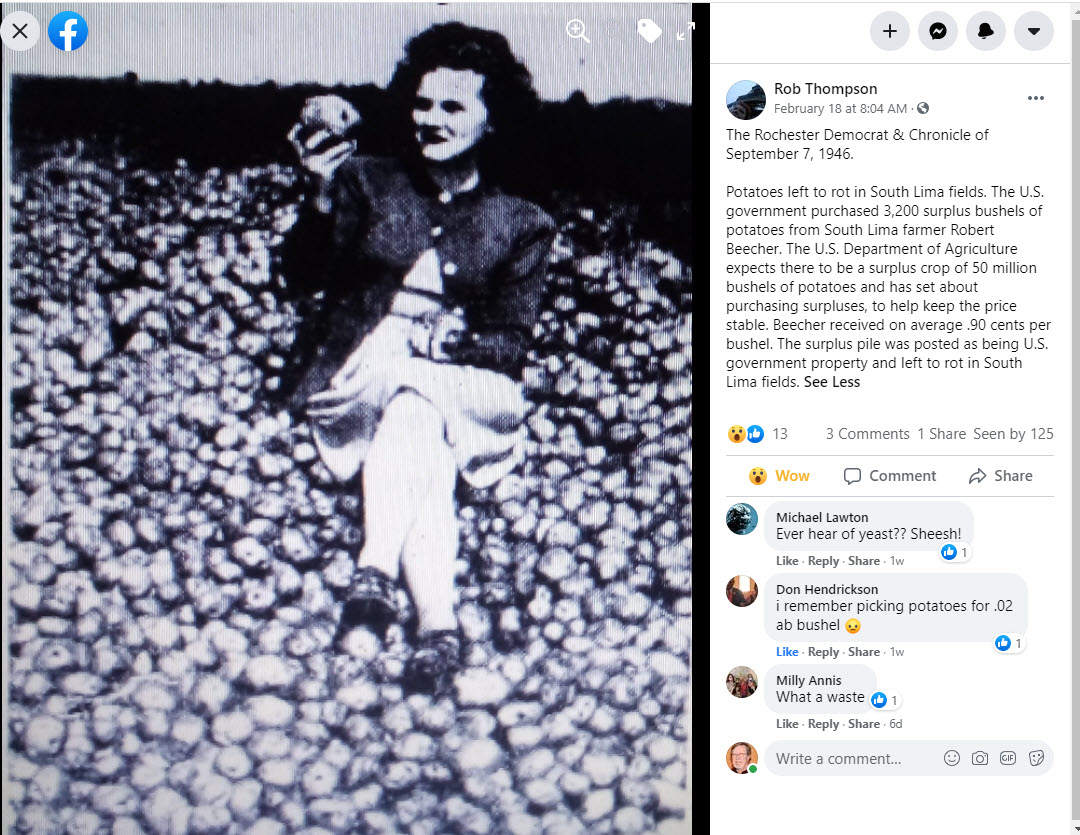The screenshot captures a Facebook post made by Rob Thompson on February 18th at 8:04 a.m. The post features an archival black-and-white photo of a young woman sitting atop a large pile of potatoes. She is dressed in a skirt, shoes, and a buttoned cardigan with short, curled hair. On the right side of the image, text provides context from an article in the Rochester Democrat and Chronicle dated September 7, 1946, detailing how the U.S. government purchased 3,200 surplus bushels of potatoes from South Lima farmer Robert Beecher. The Department of Agriculture anticipated a surplus of 50 million bushels of potatoes and bought these excesses to stabilize prices. Beecher was compensated an average of 90 cents per bushel. Despite the purchase, the surplus potatoes were designated as U.S. government property and left to rot in the fields of South Lima. The post has 13 reactions, three comments, and one share, with comments noting historical memories and expressing dismay at the waste.